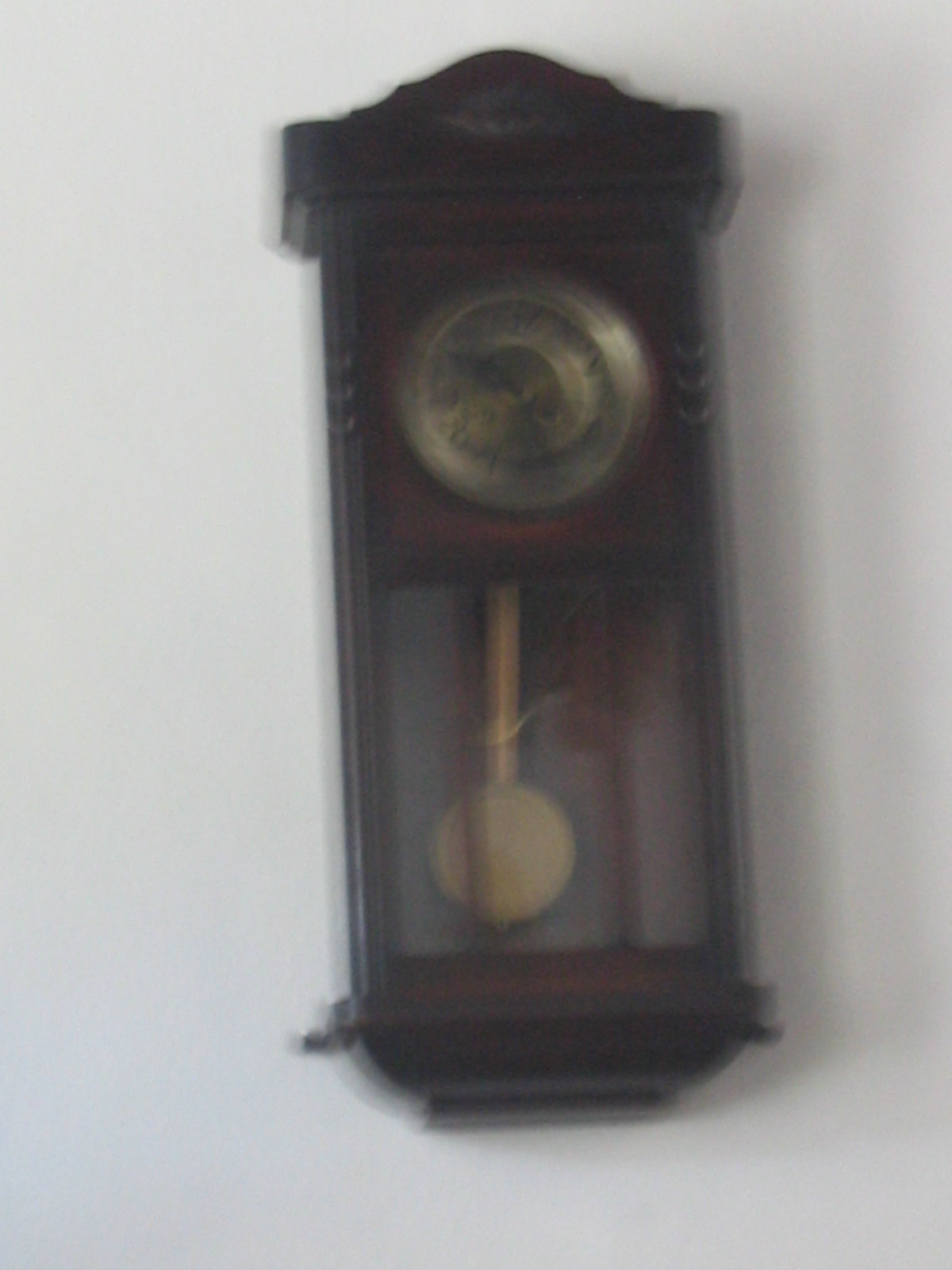This image showcases a small, wall-mounted clock designed to resemble a miniature grandfather clock. The clock is constructed from dark wood, possibly oak or walnut, and hangs against an off-white or light gray wall. The structure of the clock is tall and rectangular with a detailed top that arches outward before tapering down along the sides.

The clock face, circular and golden, appears to be made of a brass or copper material. Below the face, within a glass-paneled section, a gold-colored pendulum swings back and forth, emphasizing the clock's traditional design. The pendulum consists of a long rod with a circular weight at the end. 

Due to the poor image quality, the numbers on the clock face are indistinct, and the overall image is slightly blurry, with only the basic shape and features of the clock discernible. The wooden frame is noticeably dark, almost black, and casts a faint shadow on the wall to its right, adding depth to the composition.